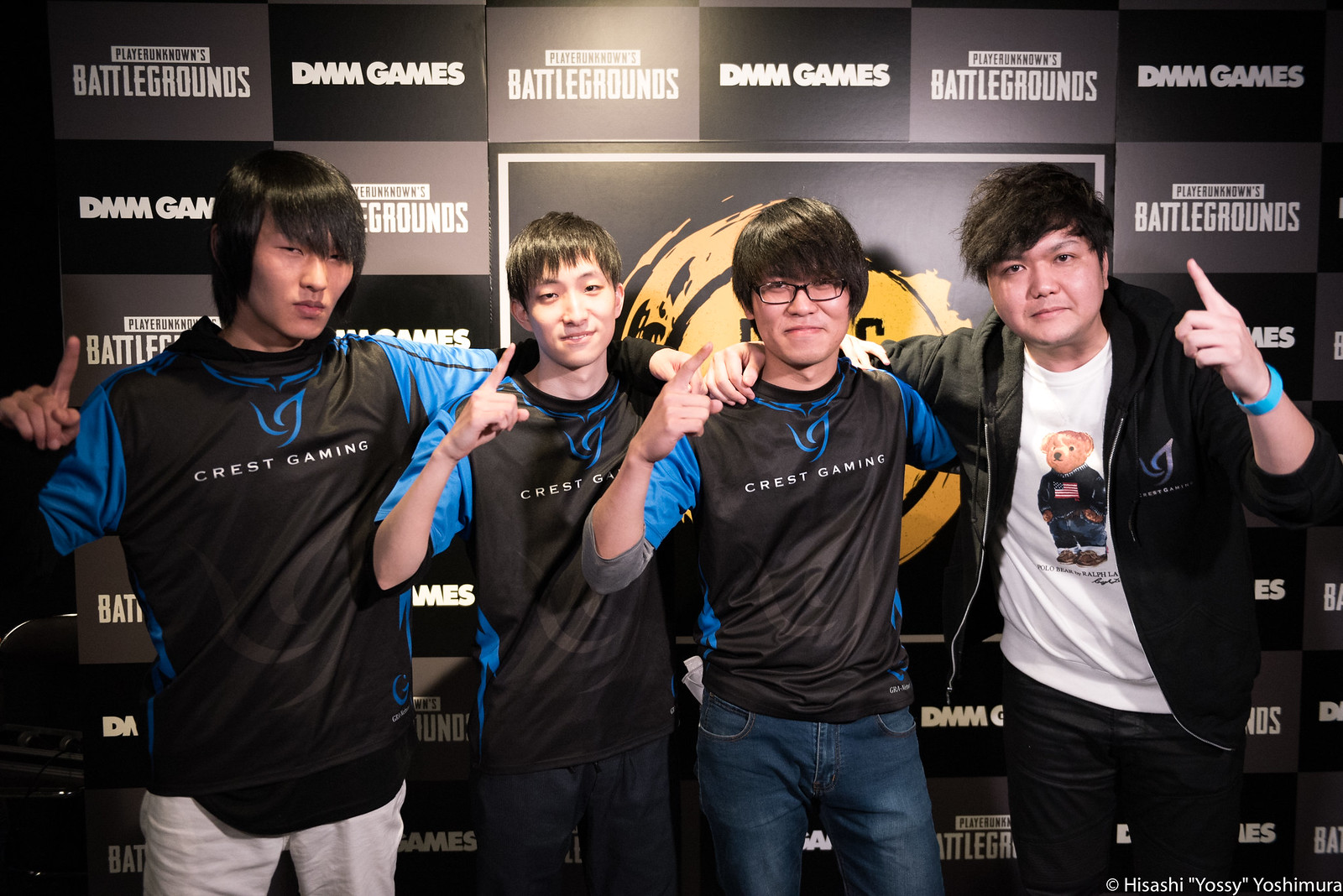Against a black background adorned with alternating rectangles that read "Player Unknowns Battlegrounds" and "DMM Games," the image prominently features four young Asian men. The backdrop includes a banner with a central gold and yellow logo, providing a visually stark canvas for the subjects. All the boys share olive skin and short black hair, contributing to a unified appearance.

Three of the boys are dressed identically in black shirts with blue sleeves and "Crest Gaming" emblazoned on the front. The boy on the far left, the tallest among them, wears white pants and sports a clean-shaven look with long hair sweeping over his forehead. His right hand is raised, pointing upward with his index finger, while his left arm is draped over the shoulder of the next boy. This second boy mirrors his pose, complete with short hair falling over his forehead and black pants.

The third boy, also following the same gesture, has medium-length hair that falls over his forehead and wears black-framed glasses with blue jeans. Their coordinated outfits and poses create a sense of unity and team spirit.

The fourth boy stands out slightly, dressed in a black hoodie jacket over a white shirt featuring a teddy bear. He pairs this with black pants and a blue wristband. His left arm rests on the shoulder of the boy next to him as he points upwards with his left hand, maintaining the uniformity of the gesture.

In the bottom right corner, the image is credited to "Hisashi 'Yoshi' Yoshi Ishimura," wrapping up this snapshot from what appears to be a gaming event.